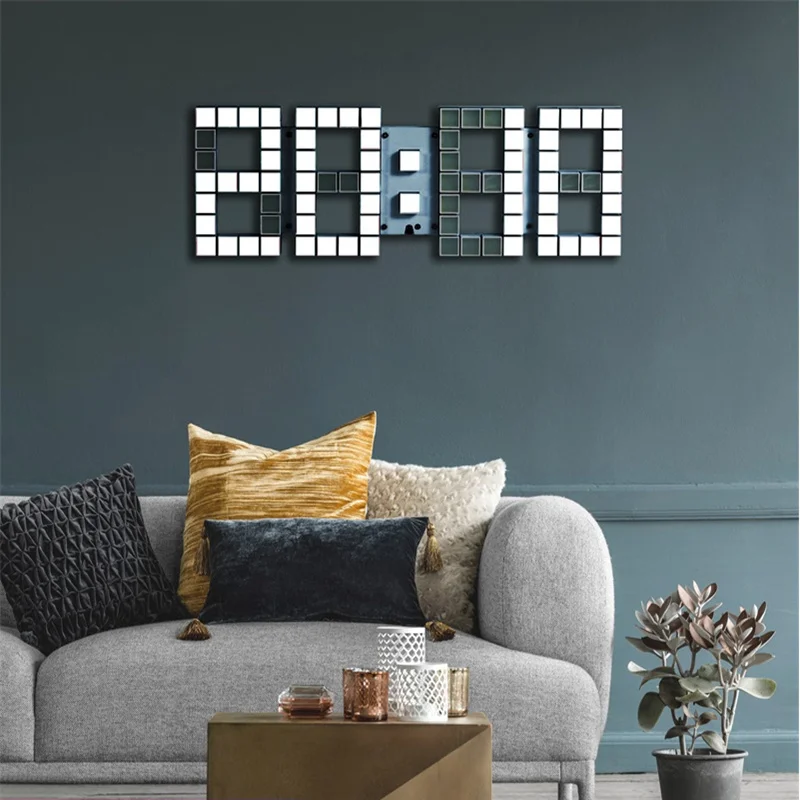This image depicts a cozy living room with a sophisticated color palette. The walls are painted in a pretty bluish-grayish hue and feature a chair rail that is the same color. Dominating one wall is a large digital clock made to blend with the wall's color, displaying the time as 20:10 (8:10 PM). Below the clock, a light gray sofa sits against the wall, adorned with four distinctive pillows: a black square pillow, a gold square pillow, a beige square pillow, and a rectangular gray pillow accented with four gold tassels. In front of the sofa, there's a brown coffee table holding several candles in varying colors and designs, including white, bronze, and gold ones. To the left of the sofa, a potted plant in a black pot adds a touch of greenery to the room. The overall composition of the room is harmonized by the consistent gray tones and accents of gold and other colors found in the pillows and decor.